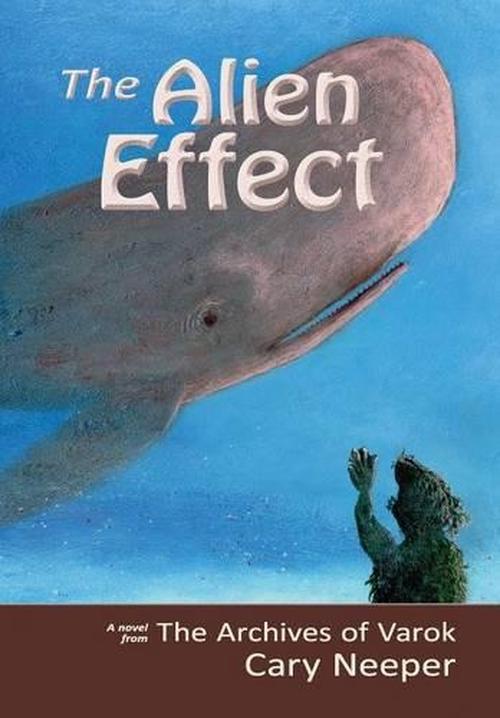The image is a book cover titled "The Alien Effect," displayed in white letters with a gray outline at the top. Dominating the upper portion is a gigantic, swimming gray whale, its front end lighter with hints of white and pink, and a dark gray back half. The open mouth and black eye are visible, suggesting it moves through a vast blue ocean. In the bottom right corner, a green creature, resembling a humanoid draped in green leaves or seaweed, raises a five-fingered arm towards the whale. At the bottom of the cover, a brown stripe holds text in white lettering that reads, "A Novel from the Archives of Varak Kari Nipper."